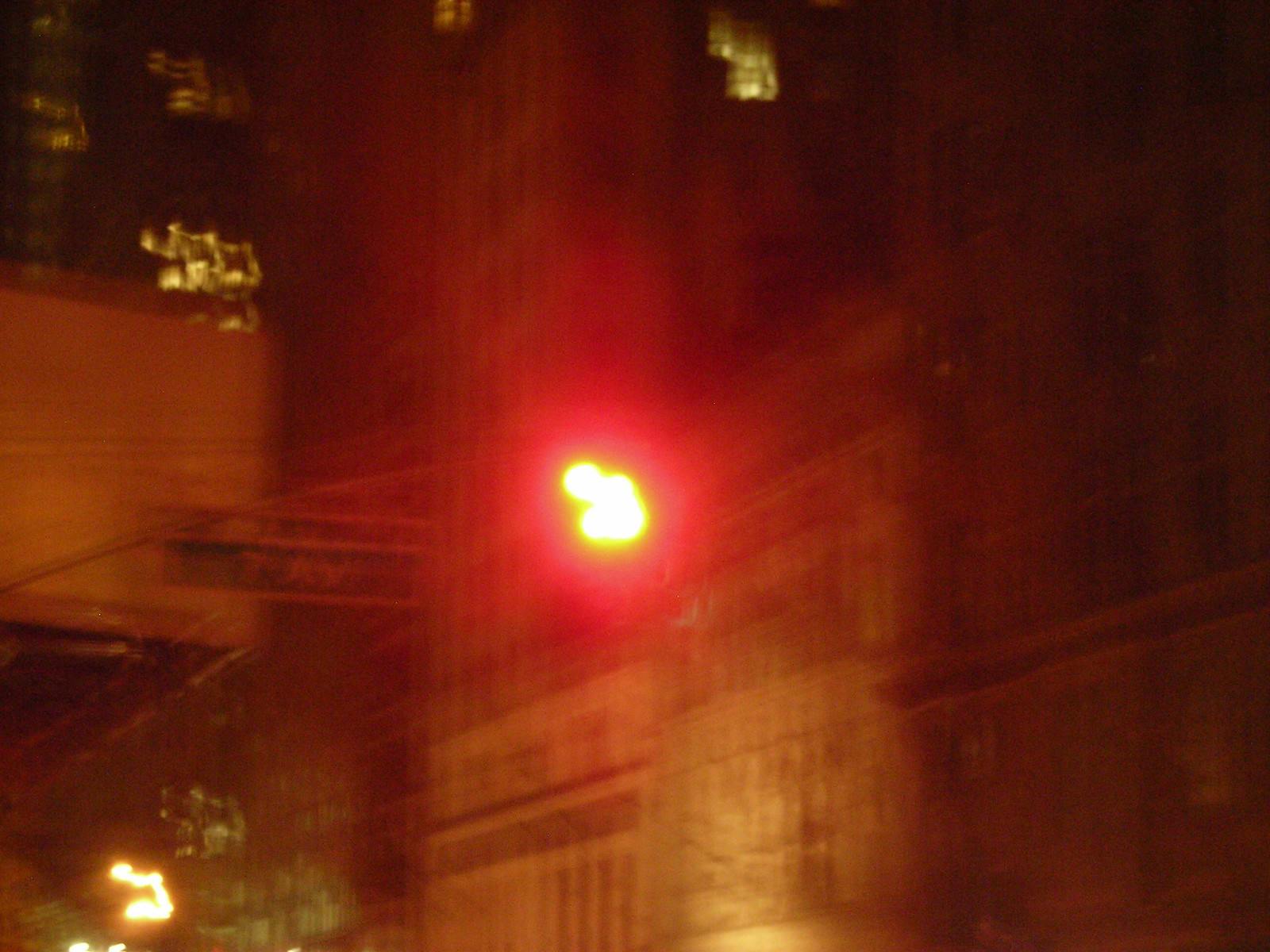A blurred nighttime image captures a city street bathed in a soft, unfocused glow. At the center, an indistinct light source casts a reddish halo, hinting at a possible streetlight or traffic signal. To the left of this light, a barely discernible street sign might indicate "7th Avenue," though the text is not clearly legible. The photograph is suffused with the ethereal silhouettes of large buildings, their faintly illuminated windows suggesting towering structures. An ambiguous, possibly indoor walkway appears on the left side of the frame, while additional high-rises loom in the distant background. The overall blur creates a dreamy, almost surreal urban landscape.